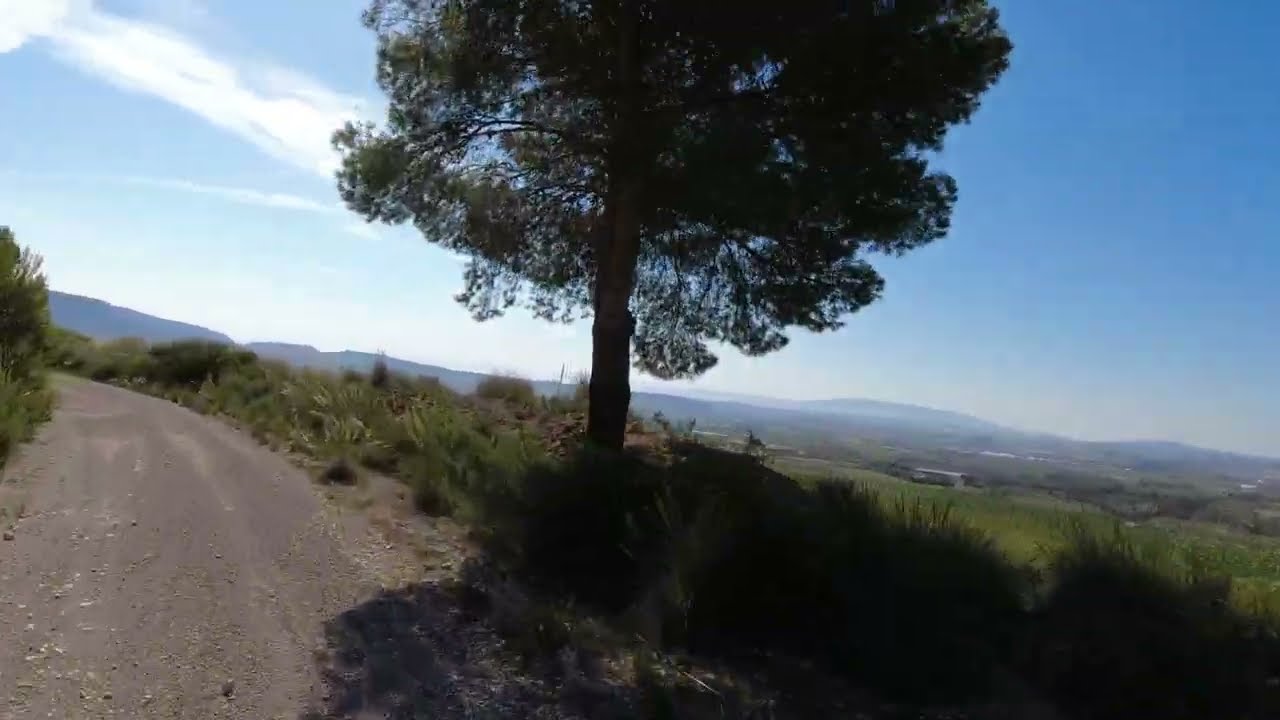This photograph, captured in a natural outdoor setting, features a winding road that begins at the bottom left and curves sharply out of view. The road's surface appears to be concrete and narrow. Prominent in the middle right of the image stands a large deciduous tree, potentially an oak, its shadow cast towards the right, indicating the sun is shining brightly. Surrounding the base of the tree and extending into the distance are lush, uncut wild grasses. On the left side of the road, additional vegetation and a smaller tree can be spotted. The landscape gradually transitions further away into a verdant valley covered in green grass. In the far distance, blue-tinted hills or a small mountain range rise on the horizon. The sky overhead is a vibrant blue with scattered white clouds, including streaks of clouds particularly visible in the top left corner. The entire scene is bathed in a soft, golden glow, suggesting either early morning or late afternoon light, enhancing the pastoral charm of the landscape. Aerial perspective implies the photograph might have been taken from a slightly elevated vantage point, possibly by a drone, offering a broad and immersive view of the serene countryside tableau.